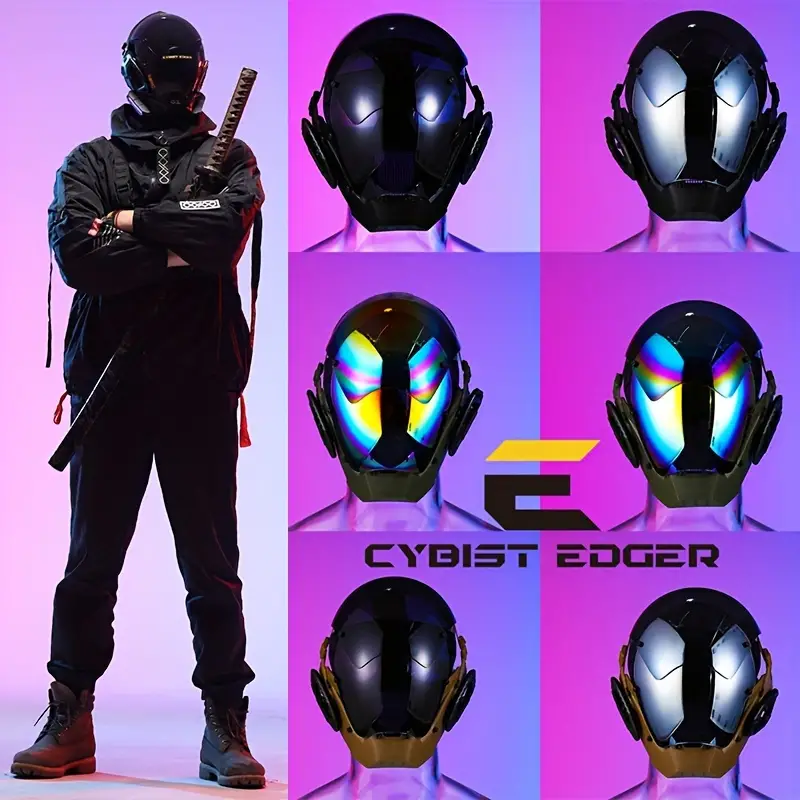In this detailed image set against a lavender to fuchsia gradient background, the left side prominently features a man in a dark, futuristic uniform. He is wearing a cybernetic helmet that obscures his face, and his apparel consists of an all-black outfit paired with brown boots. The man stands with his arms crossed, holding a large ninja sword between them, directly facing the viewer. To the right of this figure, the image is divided into three rows of two columns, displaying a total of six distinct helmets. Each helmet variation offers different aesthetics: one is completely black, another features white highlights, and others present vibrant rainbow colors that light up the helmet. The helmet style of the man on the left is also included among these variations. In the bottom right corner, one helmet is entirely silver and illuminated, adjacent to a brown one. The image contains bold text that reads "CYBEST EDGER," with an 'E' positioned above it; the top of the 'E' is yellow, transitioning into brown for the remainder.